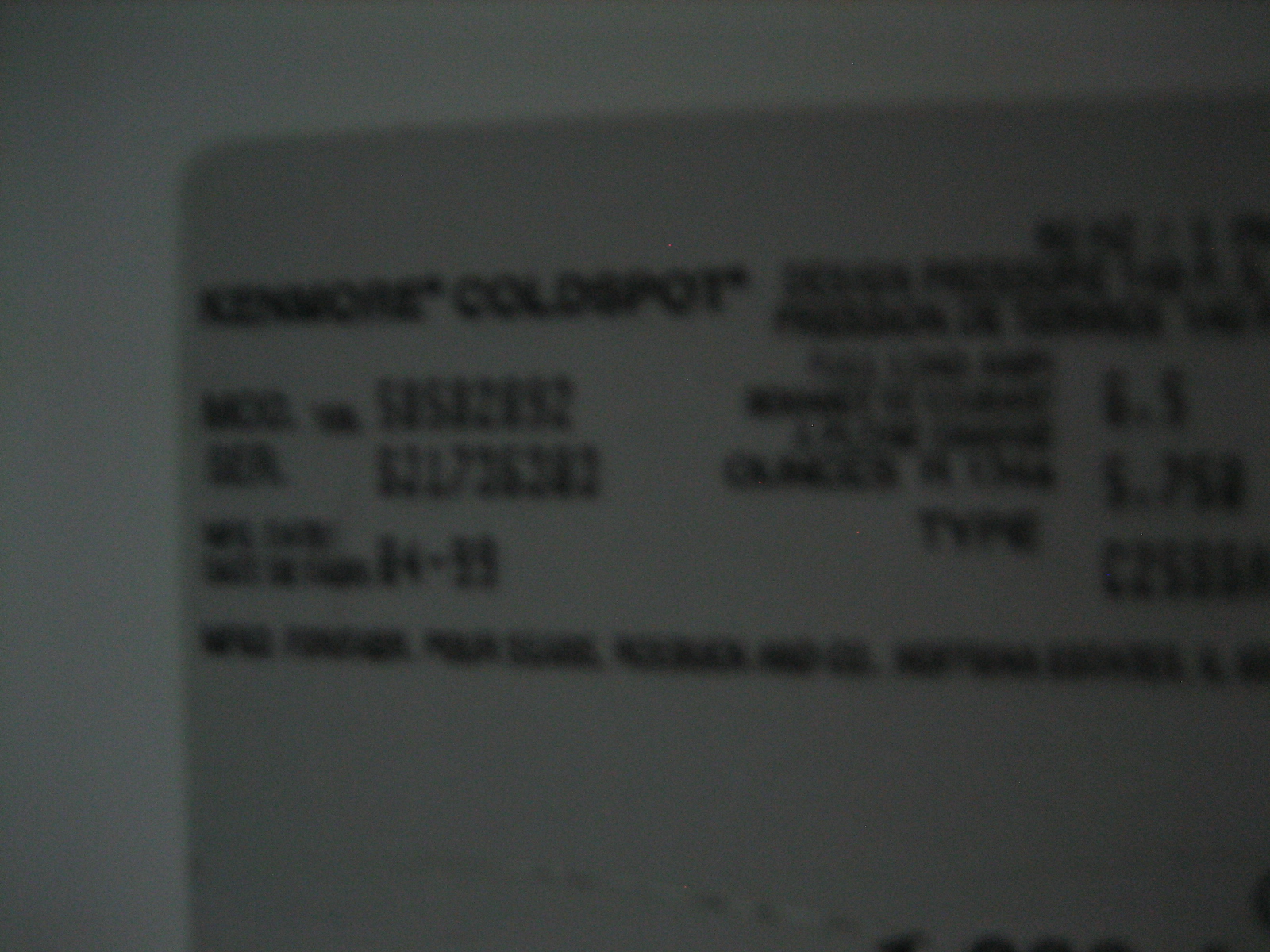Caption: The image depicts a side label on an older model refrigerator. The label, which appears slightly darker and more gray in contrast to the refrigerator's white surface, resembles a business card in its layout. Positioned horizontally from the left-hand side and extending right, it leaves about a two-inch margin at the top right corner. The label prominently displays the brand "Kenmore Cold Spot." The model number, though difficult to discern due to the blurriness, appears to be either 52582, 892, or 992. Beneath this, another number can be intermittently identified as 521726383. On the left side, the word “type” is visible, but the text at the bottom remains illegible due to the blurriness of the image.